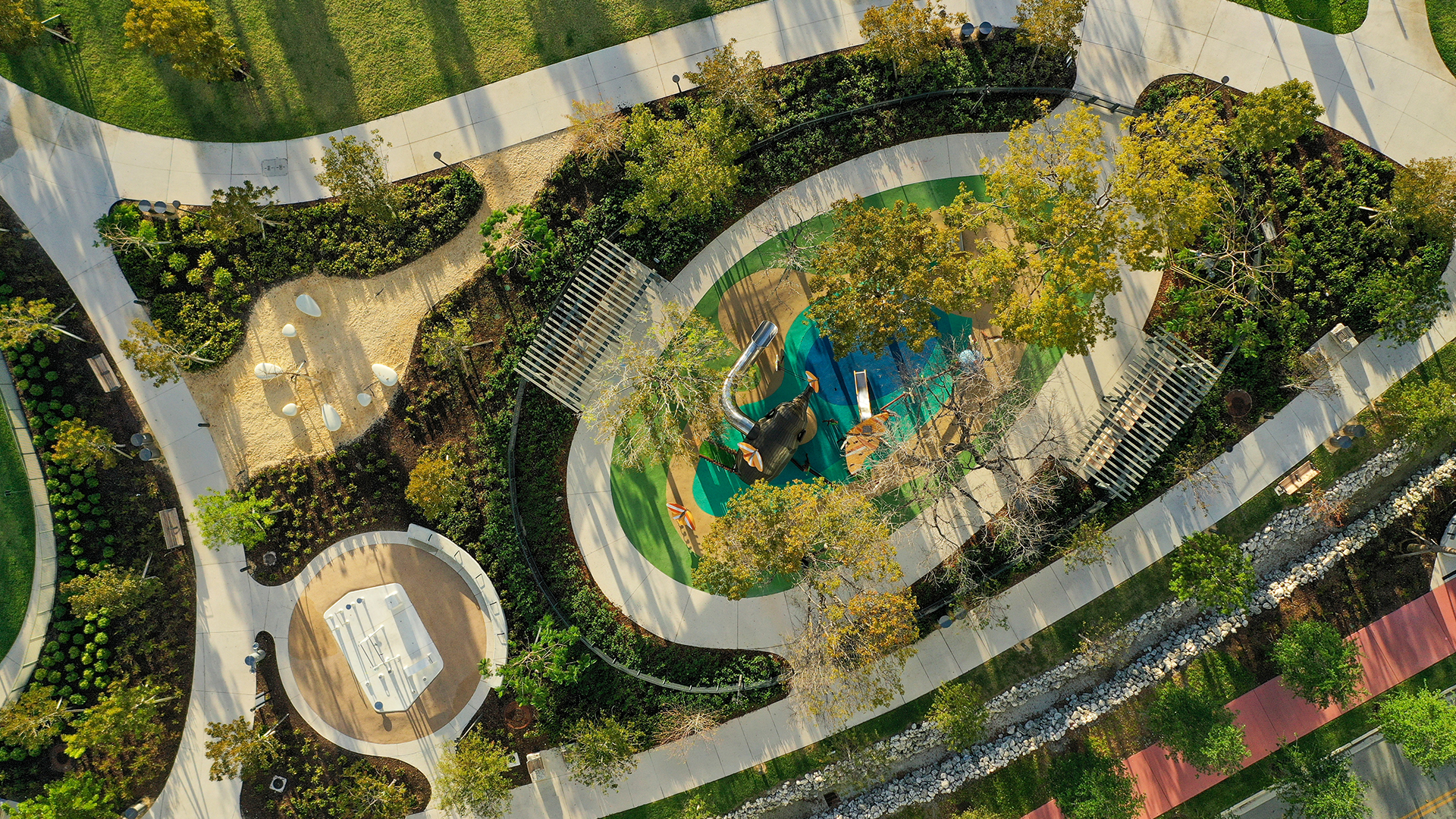This aerial photograph captures a detailed bird's eye view of a model community park that appears to be used for planning and development purposes, likely in a suburban area. The centerpiece of this park features a small body of water or pond in an oval shape, surrounded by lush green grass and numerous trees. There are multiple pathways and walkways, some of which loop around the park, offering ample space for walking. The central area includes a playground with two distinct slides—one with a black entrance and another with a yellow entrance—and patches of AstroTurf suggest that it is a child-friendly recreational area. Additionally, there are sandy or dirt areas that could be designed for various activities. The surrounding landscape is dotted with white structures that could represent buildings or houses, although their exact nature is unclear from this viewpoint. A gravel ditch for drainage is visible, and there are indications of infrastructure such as streets and possibly a stone fence, along with a red line that might signify a path or a boundary.